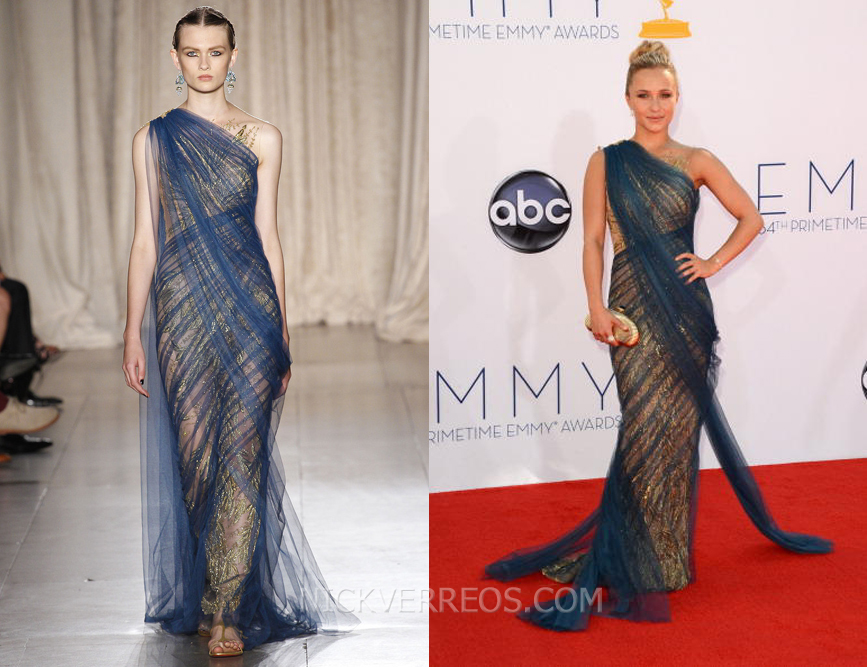The composite image features two photographs side by side. The left side shows a runway model, a white female with slicked-back hair and large blue earrings, striding confidently on a tiled floor amidst partially visible audience members. She wears a body-hugging bronze dress that appears almost nude in color, elegantly draped with a flowing sheer blue overlay, and complements her look with matching nude-colored shoes.

On the right side, a likely actress graces the red carpet, ostensibly at the Primetime Emmy Awards as indicated by the large "ABC" branding and Emmy logos on the backdrop. Clutching a small bag, she strikes a composed pose in the identical bronze dress with sheer blue overlay, her setting further contextualized by the vivid red carpet underfoot. The photo from the website is watermarked at the bottom with "nickveros.com." The image draws a striking comparison between high fashion on the runway and its glamorous translation to a major award event.